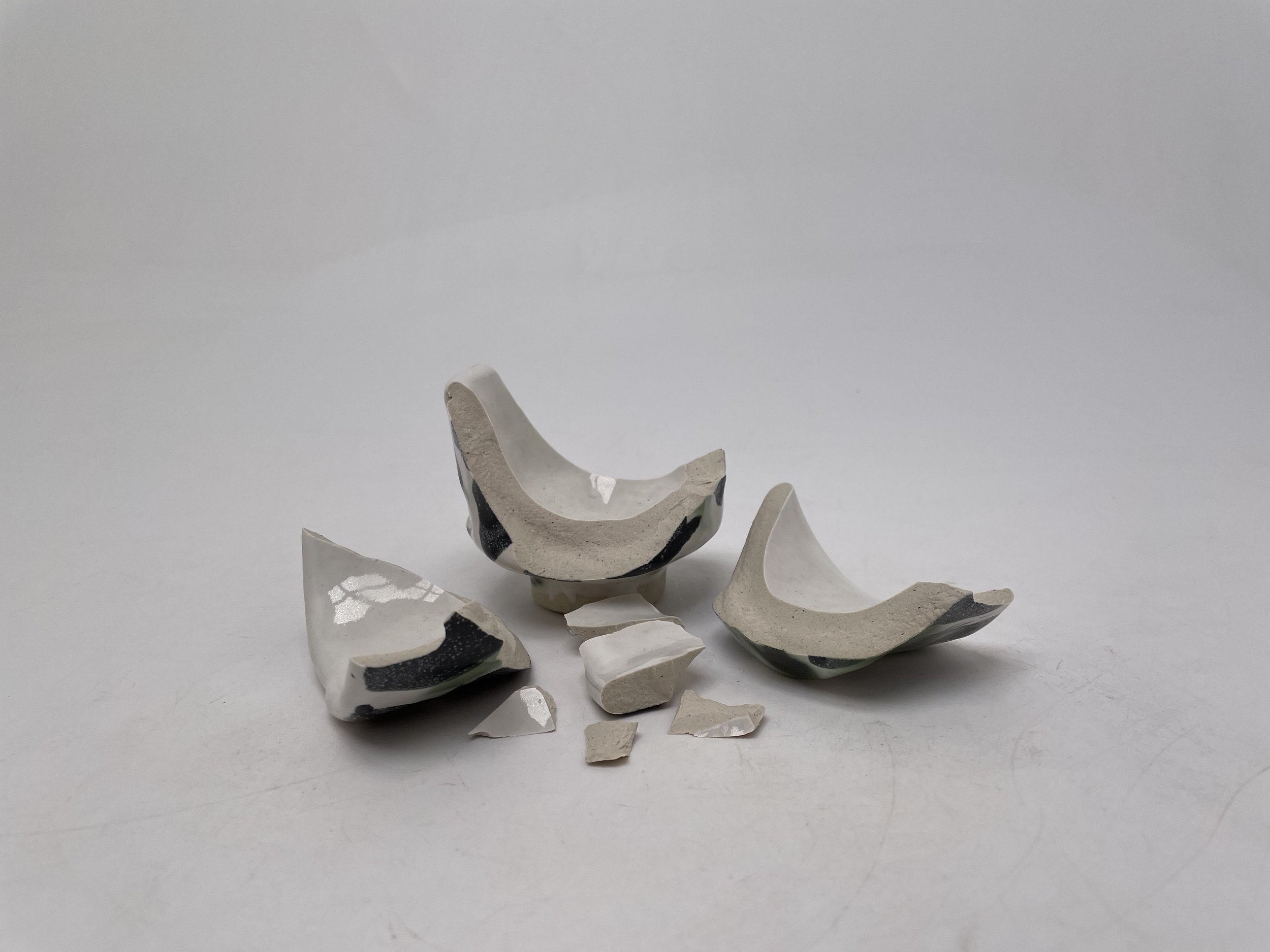The image showcases an arrangement of broken pottery at the center of a flat, light gray background. The pottery, likely old stoneware, consists of three large, gray pieces with shiny, gray enamel interiors and black stripes on the exterior, suggesting a simple yet intricate design. These major fragments are complemented by smaller chunks and thin flakes positioned among them, all boasting sharp edges that catch the light, adding a reflective gleam. Some of the pieces rest flat on their sides, while the centerpiece sits slightly upright, emphasizing the jagged, mouth-like protrusions. The background surface is uniformly gray, adorned with faint scratch lines, giving the image a clean but textured appearance. This meticulously laid-out scene highlights the fractured yet elegant aesthetics of the pottery.